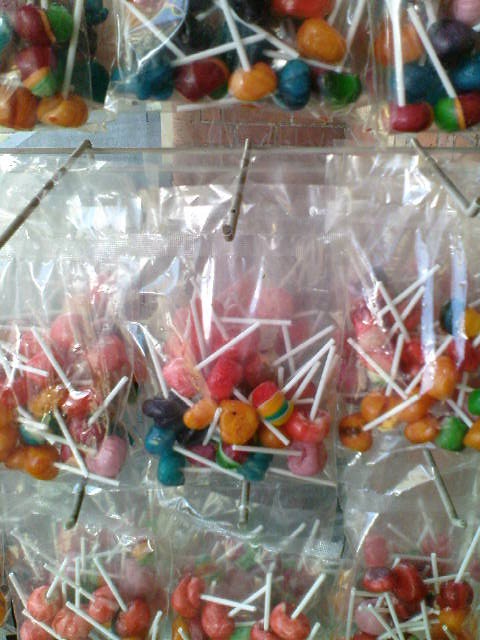The image shows a vibrant display of various colored lollipops neatly packaged in clear, plastic bags. Each bag is sealed at the top and has a small hole cut into it, allowing it to hang from thin, slightly bent metal rods protruding from a long horizontal rod that supports all the smaller rods. This layered setup features two rows of bags, each filled with lollipops that have rounded tops in a variety of colors including blue, pink, orange, dark yellow, dark green, dark blue, burgundy, and multi-colored variations of red, orange, and green. The lollipops all have distinctive white sticks. The background of the image reveals a brick wall and a sidewalk, suggesting an outdoor store display. No labeling is visible on the bags, emphasizing the candies' colorful assortment.